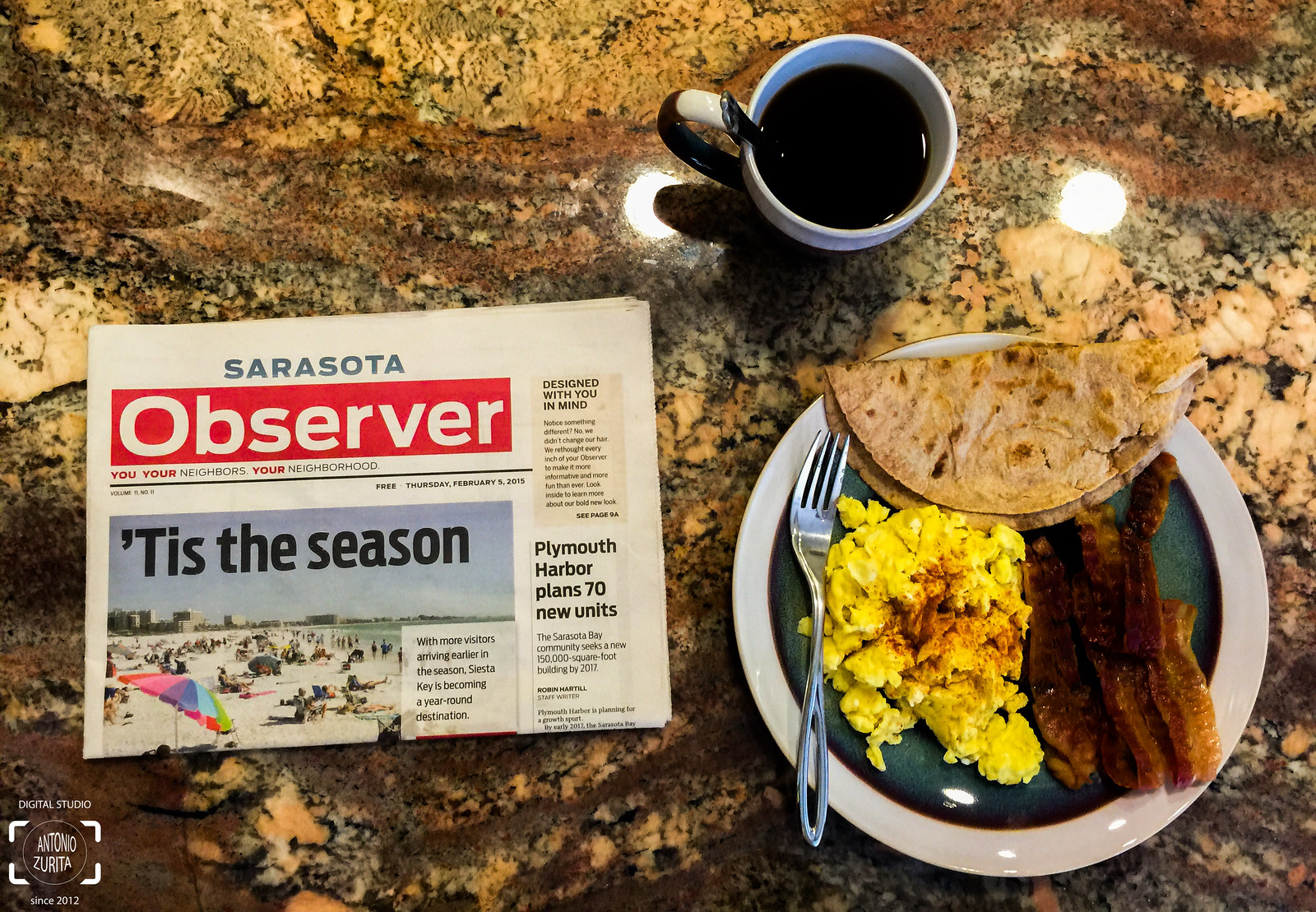In a richly detailed breakfast scene set on a polished, marbled kitchen counter with shades of brown, orange, red, and tan, a Sarasota Observer newspaper lies open, showcasing the headline "'Tis the Season" and an article about Plymouth Harbor planning 70 new units. The scene is illuminated by overhead lights reflecting off the smooth surface, which resembles petrified wood and adds a warm glow to the setting. The white-rimmed coffee cup brimming with dark coffee sits in the background, while a white plate with a dark green interior is in the foreground. The plate is arranged with a tortilla, a pile of seasoned scrambled eggs, and several strips of bacon, accompanied by a neatly placed fork. Across the bottom corner of the image, the photographer’s watermark reads "Antonio Zurita, Digital Studio," confirming the professional and artistic nature of the setup.